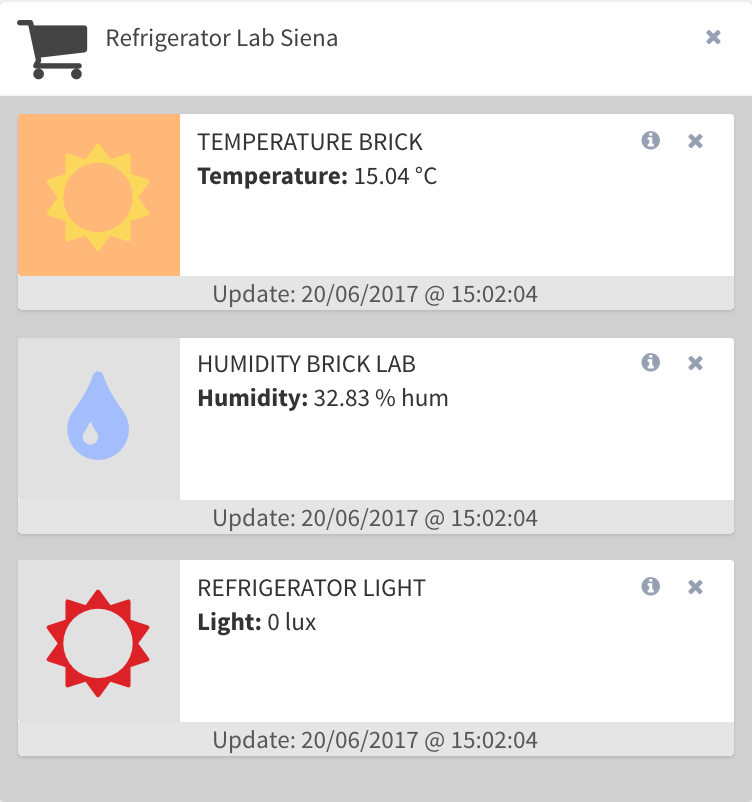The image depicts a user interface for monitoring a refrigerator, with detailed status indicators for different environmental parameters. At the top-left corner of the screen, there's a grey shopping trolley icon next to the text "Refrigerator Lab Sienna." On the top-right corner, a small 'X' is visible. Below this header, three distinct rectangular panels set against a grey background provide specific data:

1. The first panel features an orange square with a sun icon, labeled "Temperature Brick." It displays a temperature reading of 15.04 degrees Celsius, with the last update recorded on June 20th, 2017.
2. The second panel, marked with a blue droplet icon, is labeled "Humidity Brick Lab." It shows a humidity level of 32.83%, also last updated on June 20th, 2017.
3. The third panel contains a red circular icon resembling a sun with a rectangular pattern around its edge. This panel is labeled "Refrigerator Light," indicating a light level of 0 lux, with the update date similarly noted as June 20th, 2017.

Each panel is distinctly colored and iconically marked to clearly convey the status of the refrigerator's temperature, humidity, and light conditions.